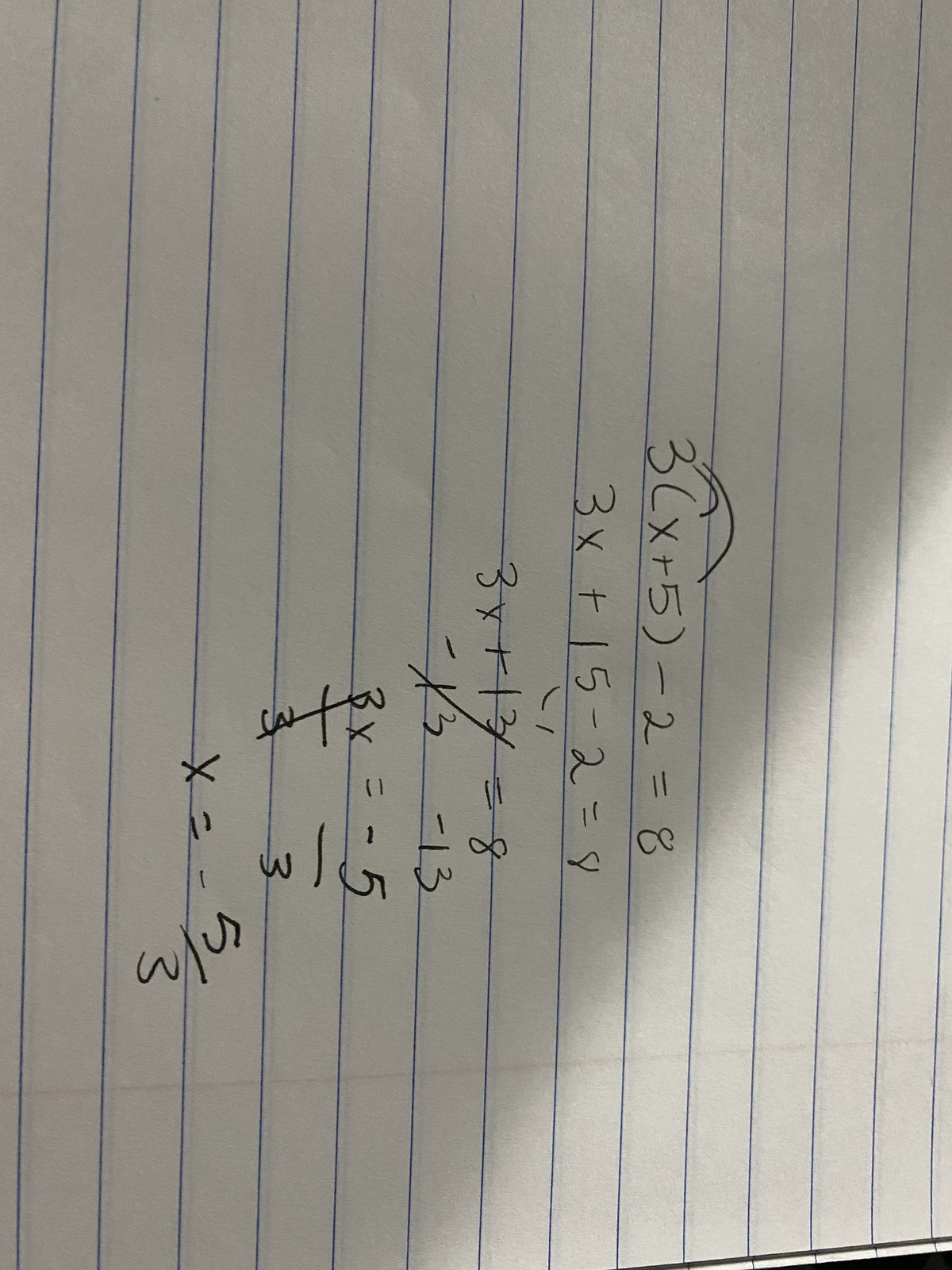The image displays a step-by-step solution to a basic algebra problem on college-ruled paper, although the picture is rotated 90 degrees clockwise. The problem begins with the equation \(3(x + 5) - 2 = 8\). The steps shown are as follows:

1. Distribute the 3, resulting in \(3x + 15 - 2 = 8\).
2. Simplify the expression to \(3x + 13 = 8\).
3. Subtract 13 from both sides to get \(3x = -5\).
4. Finally, divide by 3 on both sides to find \(x = \frac{-5}{3}\).

This descriptive sequence captures the process of solving for x in a detailed manner.